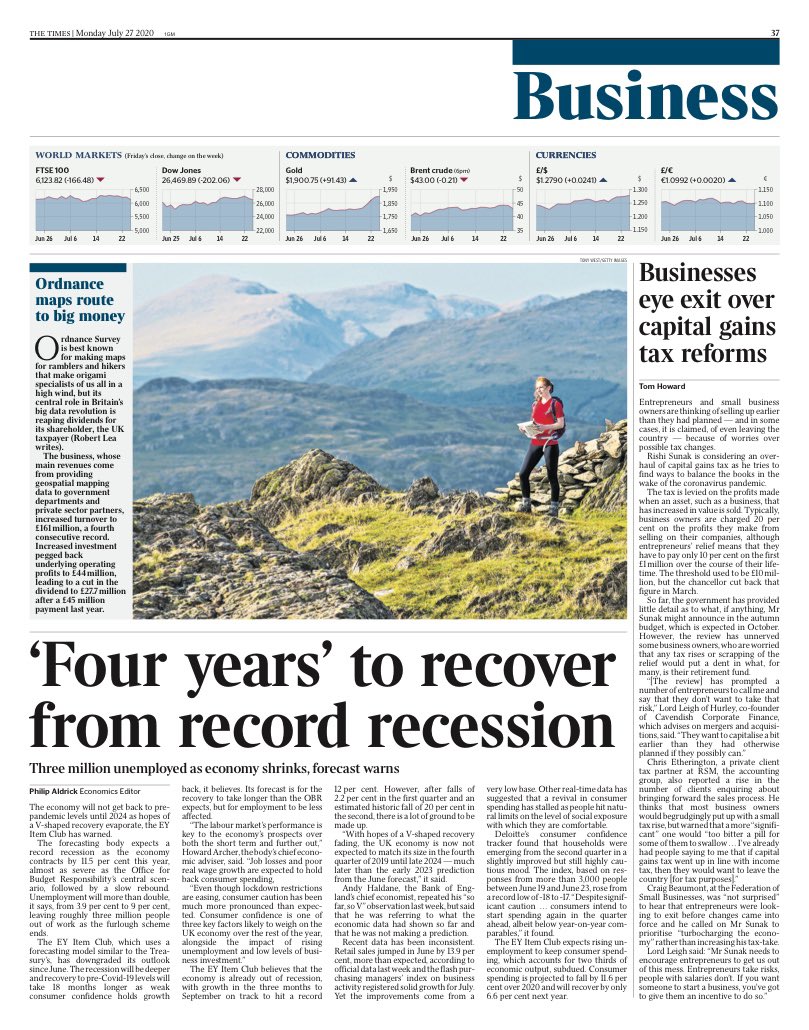Screenshot of an online newspaper page dated Monday, July 27, 2020. It is from the Business section, identifiable by a medium navy blue banner in the upper right-hand corner with the word “Business.” The top portion of the page features current data on global markets, including indices such as the FTSE and Dow Jones, alongside commodities like gold and crude oil, and comparisons of currencies, specifically between the pound, dollar, and euro.

Prominently displayed is an article titled "Four years to recover from record recession," highlighting that three million people are unemployed as the economy contracts, with forecasts warning of a prolonged recovery period. The accompanying image shows a person at the summit of a mountain, holding a book or papers and appearing triumphant, dressed in a red shirt.

Two additional articles are sectioned below. One is titled "Ordinance maps route to big money," and the other addresses a contentious issue with the headline "Businesses eye exit over capital gains tax reform," indicating companies' plans to navigate through impending tax changes.